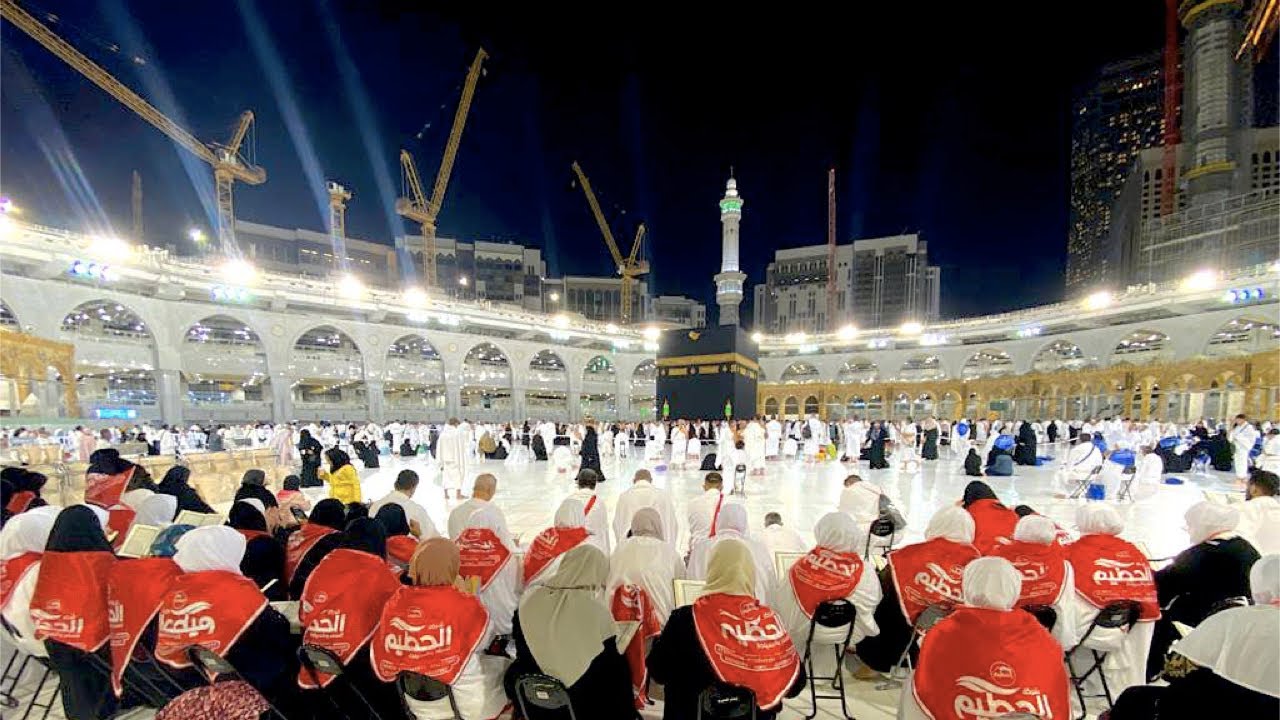The image depicts a reverential scene within the open-air area of the Kaaba in Mecca, the focal point of the Islamic faith. Bathed in the glow of bright lights that illuminate the sacred space, hundreds of people are seen both sitting and standing, many bowing their heads in reverence and prayer on a floor that appears almost white, reminiscent of ice. The worshippers in the foreground wear headscarves and red shawls featuring Arabic script, and they face away from the viewer towards the Kaaba, the large black stone structure at the center of the arena. The surrounding architecture includes intricate arches and columns that encircle the perimeter, opening directly up to a dark nighttime sky dotted with towering office buildings and skyscrapers. The scene captures the ongoing construction with numerous cranes visible on the left side, while the multi-story walls with semicircular arches create a blend of ancient reverence and modern urban backdrop.